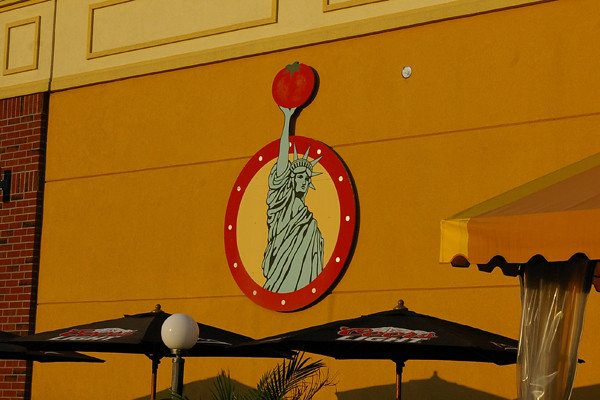This image captures a colorful and eclectic scene outside a restaurant. Dominating the center of the composition is a circular medallion mounted on an orange wall. The medallion features a cartoon depiction of the Statue of Liberty holding a tomato aloft in her right hand, set against a yellow background and encircled by a red border with white polka dots. To the left of the wall is a brick building with yellow and gold paneling above it. Guarding this charming tableau below are black umbrellas emblazoned with the Coors Light logo. Additional details include the top of a green plant, part of a light post, and another umbrella. The scene's vivid colors and quirky elements create an inviting and vibrant atmosphere.